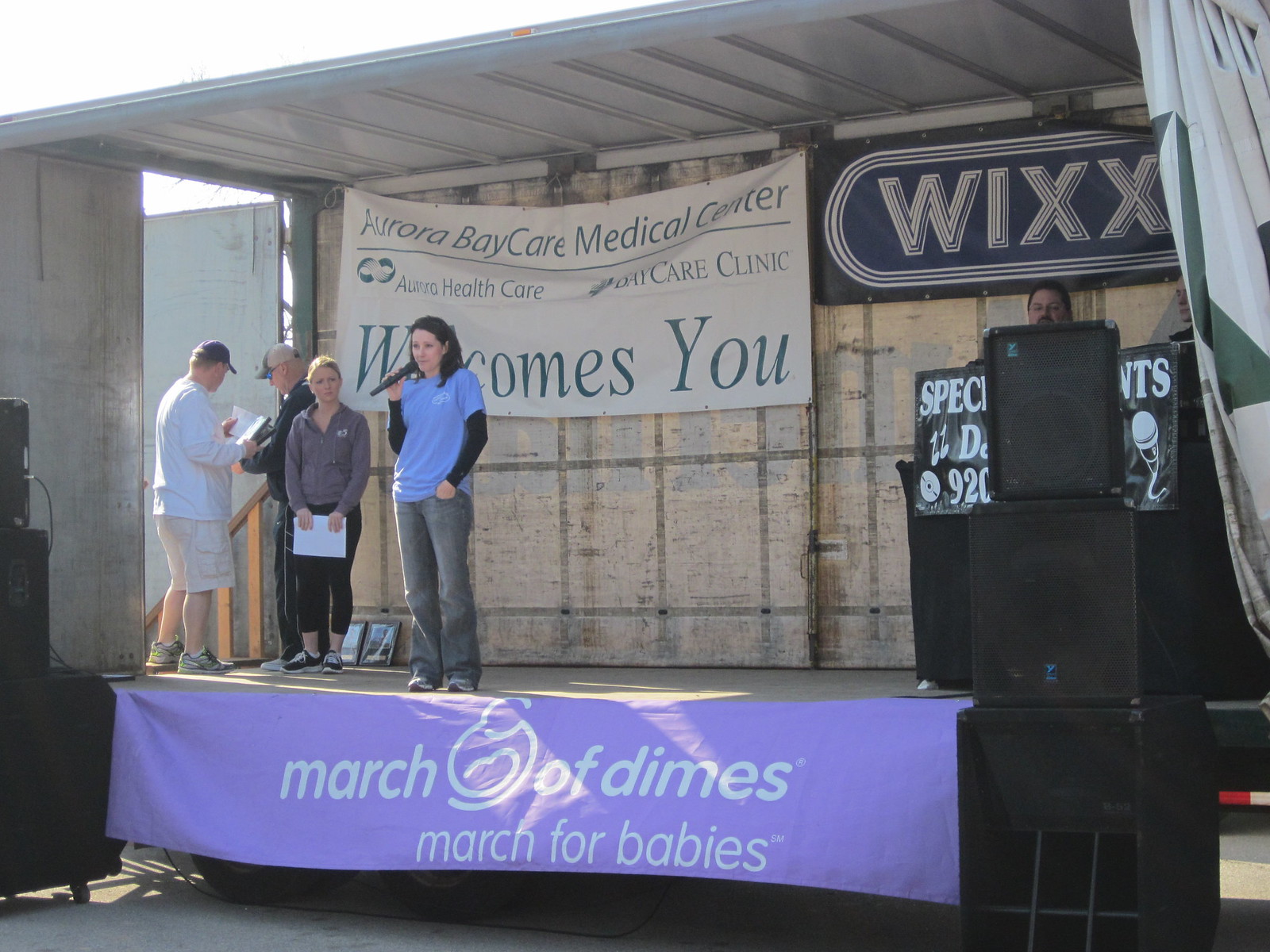In this photograph, a woman stands on an outdoor stage holding a microphone to her mouth. She is dressed in a light blue t-shirt over a black long-sleeved shirt and jeans. The woman, who has black hair and a fair complexion, is seemingly addressing an audience as part of an event. To her left, another woman wearing a gray sweatshirt holds onto what appears to be a prepared speech. Behind the second woman, two older men are engaged in conversation. The stage is adorned with a banner at its base reading "March of Dimes, March for Babies." Behind the speaker, another banner is prominently displayed stating "Aurora Bay Care Medical Center, Aurora Health Care, Bay Care Clinic, welcomes you." Additionally, a sign for WIXX is visible in the background. The stage is equipped with multiple speakers, contributing to the event's professional setup.